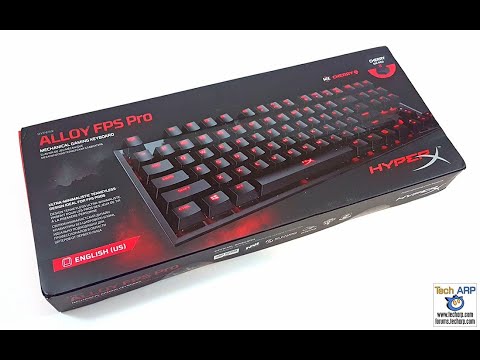This image features a screenshot of a keyboard in its original packaging with a predominantly white background. Two black stripes run horizontally across the top and bottom of the image. The product packaging itself is a long rectangular black box with a durable appearance. Prominently displayed on the front cover is the keyboard, which features illuminated red keys. The product name, "Alloy FPS Pro," is highlighted in red, while a red banner at the bottom reads "English US" in white text. Additional features of the keyboard are detailed in white text on the packaging. The brand name, HyperX, is cleverly designed with "Hyper" in red and "X" in silver, located at the bottom right corner of the packaging. Adding further detail to the image, there is a small box at the bottom right corner that says "TEC ARP" with "TEC" in yellow and "ARP" in dark green, all capitalized. Accompanying this, there is a logo depicting an animal with blue fur, a white face, and two glowing eyes, along with a URL in black beneath it.